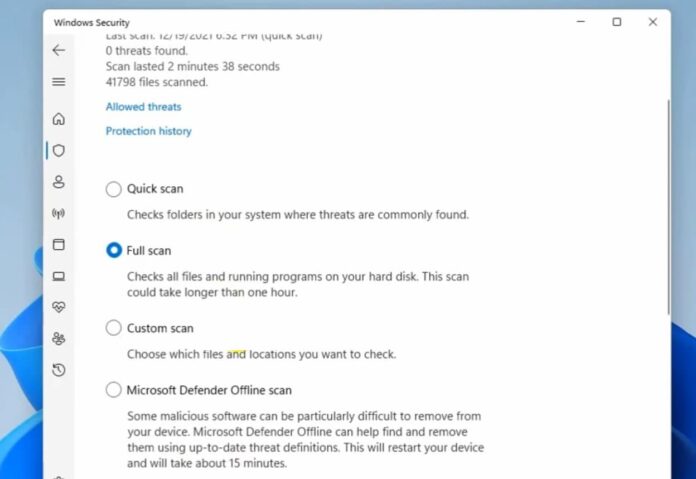The image depicts a blurry, pixelated, low-resolution screen displaying the Windows Security interface. Despite the poor image quality, details are discernible. The top-left corner of the window shows the title "Windows Security," and the top-right corner features three control buttons: Minimize, Fullscreen, and Close (X). Below the title, the interface indicates "Zero Threats Found," with the scan having taken 2 minutes and 38 seconds to complete, during which 41,798 files were scanned.

Further down, two sections are visible: "Allowed Threats" and "Protection History." Additionally, four bullet points outline different scan options. The first option, "Quick Scan," is noted to check folders in the system where threats are commonly found. The second option, "Full Scan," is described as a comprehensive check of all files and running programs on the hard disk, with a warning that it may take longer than one hour to complete.